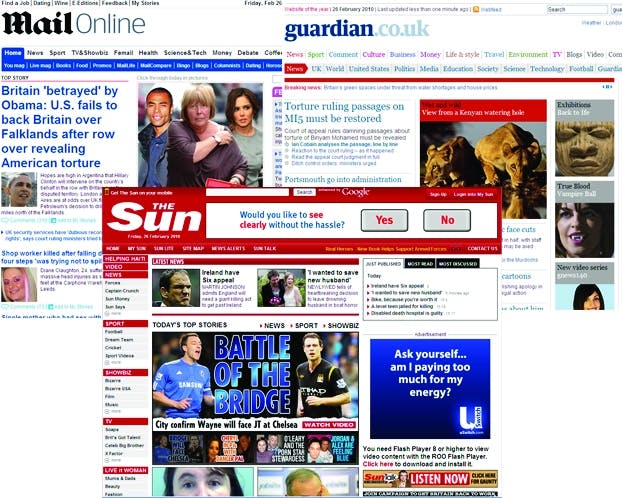The image appears to be a compilation of screenshots from various UK news publications.

The first segment is from the Mail Online. At the top of this portion, there is a series of black submenus with options like "Find a Job," "Dating," "Wine," "Feedback," and more. Below this, another menu appears with categories such as "Home," "News," "Sport," "TV & Showbiz," "Family," "Health," "Science & Tech," "Money," and "Debate." The subsequent section is a blue area with white font, which is unfortunately too blurry to read. Various headlines can be observed, including one that reads: "Britain Betrayed by Obama: U.S. Fails to Back Britain Over Falklands After Row Over Revealing American Torture," accompanied by a paragraph of text. 

Another portion of the image is from The Guardian's website, recognizable by the submenus in different colors: pink, blue, orange, and green. Categories like "News," "Sport," "Comment," "Culture," "Money," "Life & Style," and "Entertainment" are listed here. The submenu offers further options such as "News," "UK," "World," "United States," "Politics," "Media," "Education," "Society," "Science," "Technology," and "Football." A visible headline in this section reads, "Torture Ruling: Passengers on MI5 Must Be Restored," with images of lions and other visuals partially cut off. One of the images shows a piece of artwork, while another displays a scene from "True Blood," featuring a woman with vampire fangs.

Lastly, there is a segment from The Sun's website. A pop-up ad on this page asks, "Would you like to see clearly without the hassle?" with options to respond "Yes" or "No." The overall design of this segment is predominantly red and white. Prominent headlines like "Battle at the Bridge" can be seen, alongside images of sports players and various other headlines and ads. 

In summary, the image is a detailed collage of screen grabs from multiple UK news sites, showcasing their different layouts, submenu options, and headlines on diverse topics.